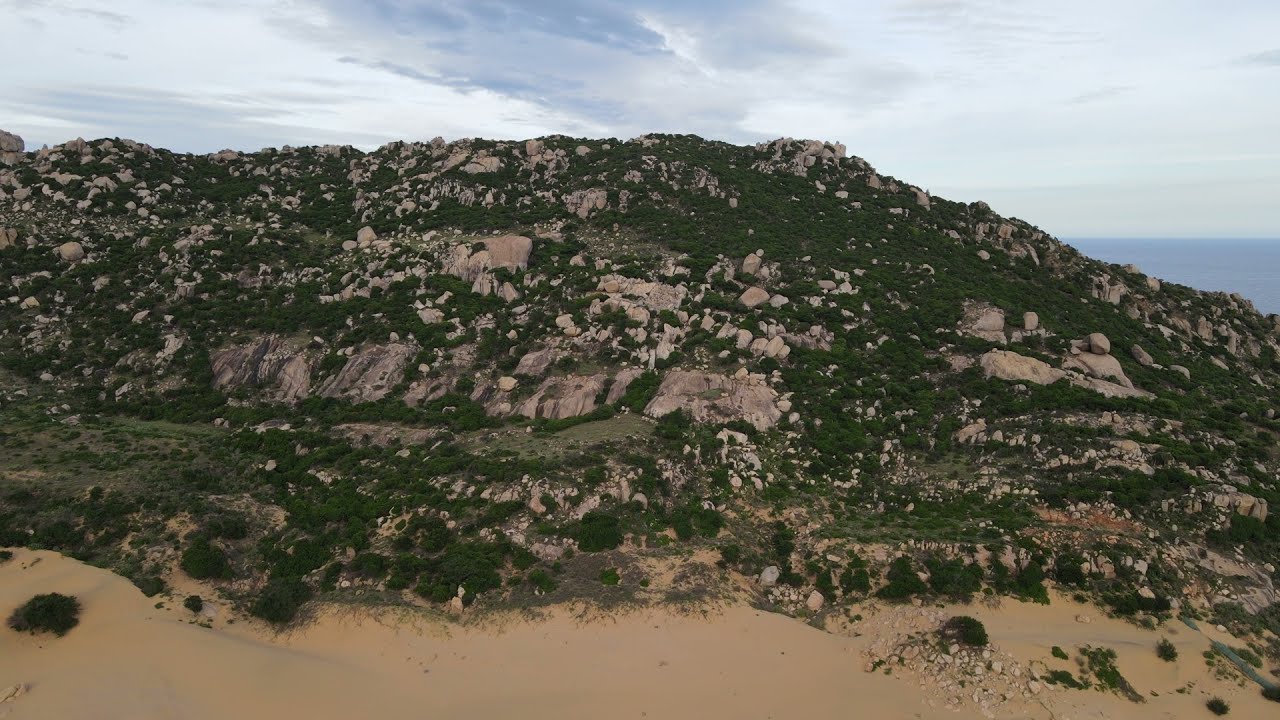This photograph captures a large, bumpy hillside covered in small green shrubs and bushes interspersed with numerous beige and gray rocks. The foreground features a sandy beige area, likely transitioning into the base of the hill. The sky overhead appears partially cloudy, with a light blue hue and patches of grayish clouds, giving a slightly overcast atmosphere. In the background, a body of water, possibly an ocean, can be seen, enhancing the impression of an outdoor, coastal environment. The scenic view appears to be devoid of people and animals, emphasizing the natural and undisturbed landscape.